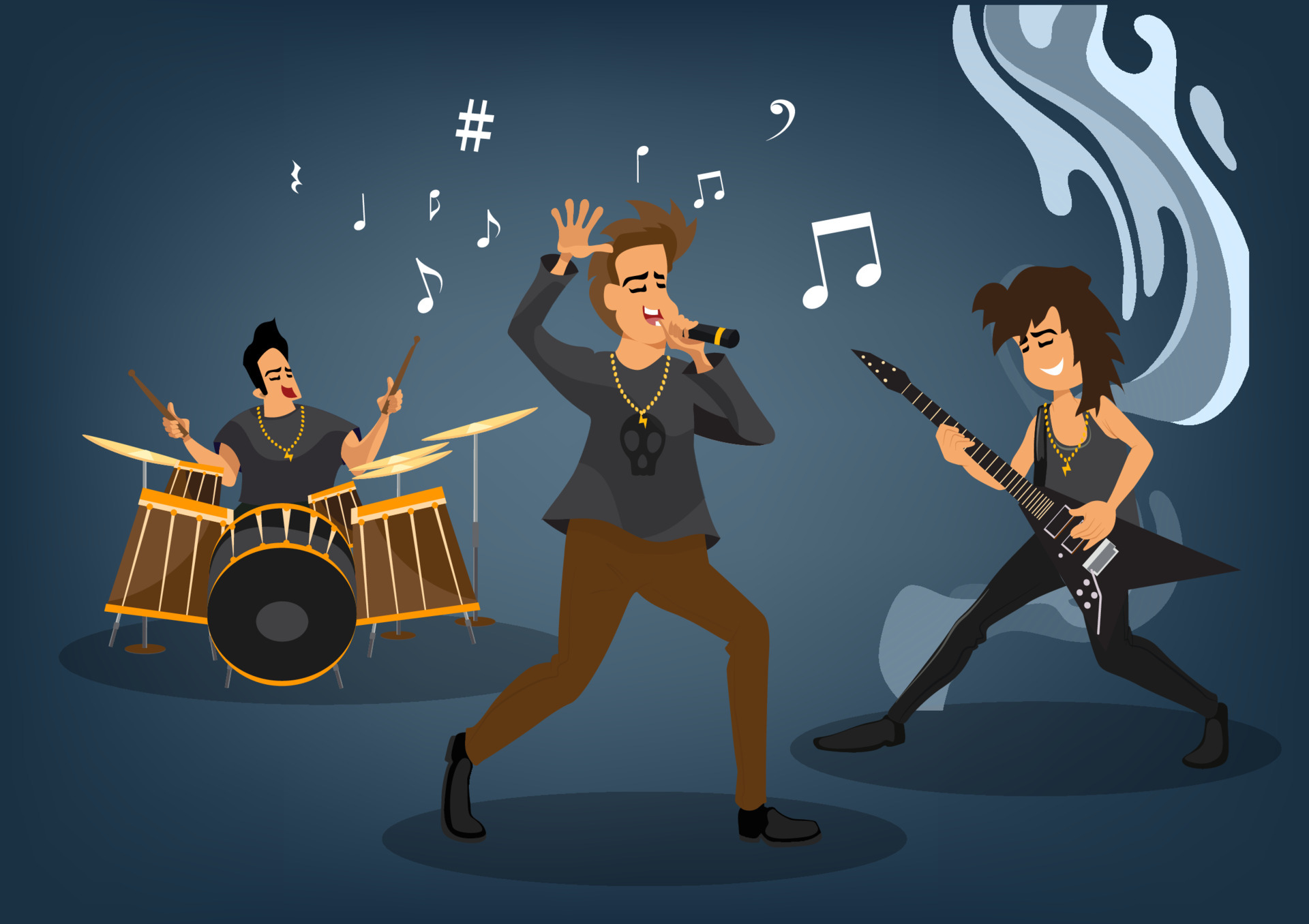This vividly colored illustration, reminiscent of the classic Hanna-Barbera style, captures a dynamic rock band in full performance mode. On the left, the drummer, adorned with remarkably red lips and a short, slightly pompadour-style dark hair, passionately plays a drum kit consisting of a black bass drum with yellow and orange accents, four smaller drums with dark brown and orange elements, and gold cymbals. He wields brown drumsticks and wears a dark t-shirt, along with a distinctive gold chain featuring a yellow lightning bolt. Central in the composition is the energetic lead singer, identifiable by a dark gray long sleeve shirt emblazoned with a black skull, skinny brown pants, and black shoes. The singer, also accessorized with the signature lightning bolt necklace, grips the microphone with his left hand while raising his right hand, and is surrounded by a flurry of musical notes, flats, sharps, and other musical symbols floating in the air against the dark gray background. To the right stands the guitar player, a woman with brown hair and closed eyes, smiling with clenched teeth as she strums a predominantly black V-shaped guitar with white accents. She is dressed in a gray tank top, skinny black pants, and black shoes, and also wears the matching gold chain with the yellow lightning bolt pendant. A stylized, swirling grayish blue pattern emanates behind her, adding a sense of motion and energy to the vibrant scene.